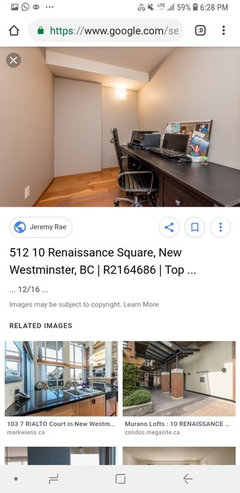The screenshot depicts a Google search performed on a smartphone, as evidenced by the portrait orientation and the typical icons along the top of the screen. On the right side of the status bar, the time is shown as 6:28 PM, alongside battery and network indicators displaying 59% charge and signal strength. The left side of the status bar contains additional standard icons.

Beneath the status bar, the search bar displays the URL "https://www.google.com/.se," with the HTTPS in green and a padlock icon indicating a secure connection. To the left of the URL is a home button icon.

The main content of the screenshot is a photograph of a room, likely an office or workspace. The room features a black wooden desk positioned to the right, paired with a matching black desk chair. A white door is located on the wall directly facing the viewer. Below the photograph, the name "Jeremy Ray" is accompanied by a small globe icon, suggesting this is a website link. The address "51210 Renaissance Square, New Westminster, BC, R2164686" follows, possibly indicating a location in British Columbia. The term "top" might imply this is a top-floor apartment or office.

Text below the address reads "12 out of 16," likely denoting that this image is the 12th in a series of 16 images. There is also a standard note that images may be subject to copyright, with a link to "Learn more." Additionally, there are thumbnails of related images, which appear to showcase similar office spaces, hinting that these might be offices available for rent in British Columbia.